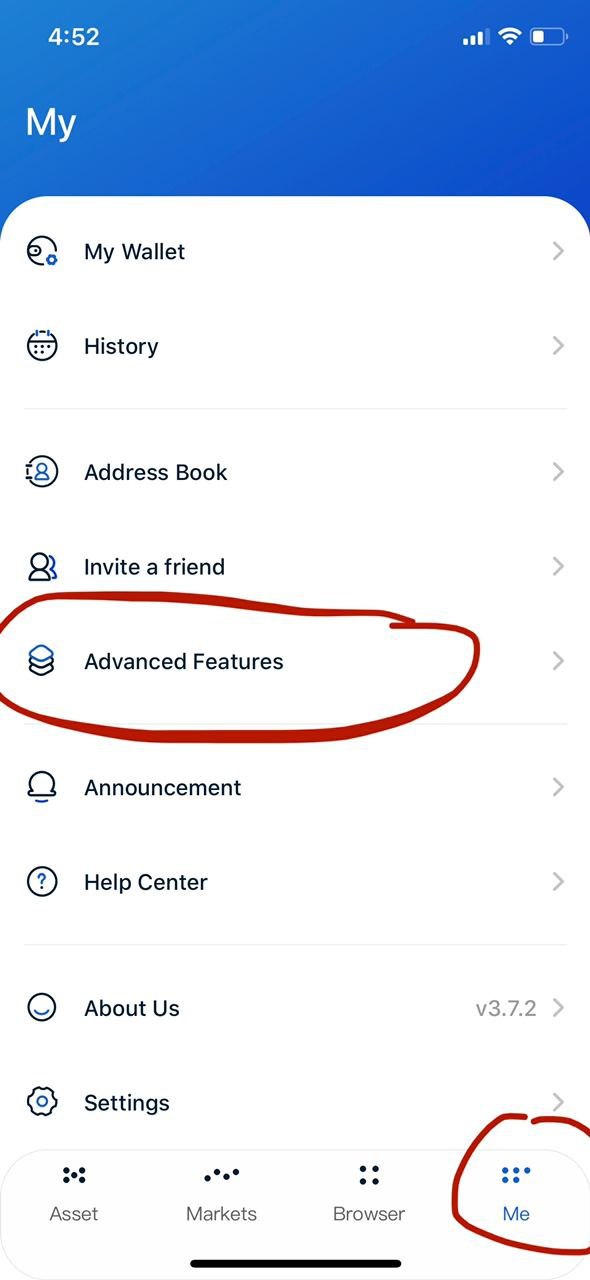This is a detailed screenshot of a mobile app interface, presented on a phone. At the top, a blue status bar spans across the screen, displaying various indicators: the time on the left shows 4:52, while the right side features icons for the phone signal, internet connection, and a battery icon, which appears to be approximately one-third full. In the center of this blue bar, the word "my" is prominently displayed in white font.

The main content of the screenshot is set against a clean white background, with various options listed in black text. Each option represents a clickable link to a different page. Starting from the top, the options include: "My Wallet," "History," followed by a thin gray divider line. Next, it features "Address Book," "Invite a Friend," and "Advanced Features," with the latter circled in red for emphasis.

Below these options, further down the list, are "Announcement" and "Help Center," separated by another thin gray line. The lower portion lists "About Us," next to which the version number "v3.7.2" is mentioned. Following this, "Settings" is noted before reaching the bottom navigation bar, which provides quick access to "Asset," "Markets," "Browser," and "Me." The "Me" option is also circled in red, indicating it's currently selected or highlighted.